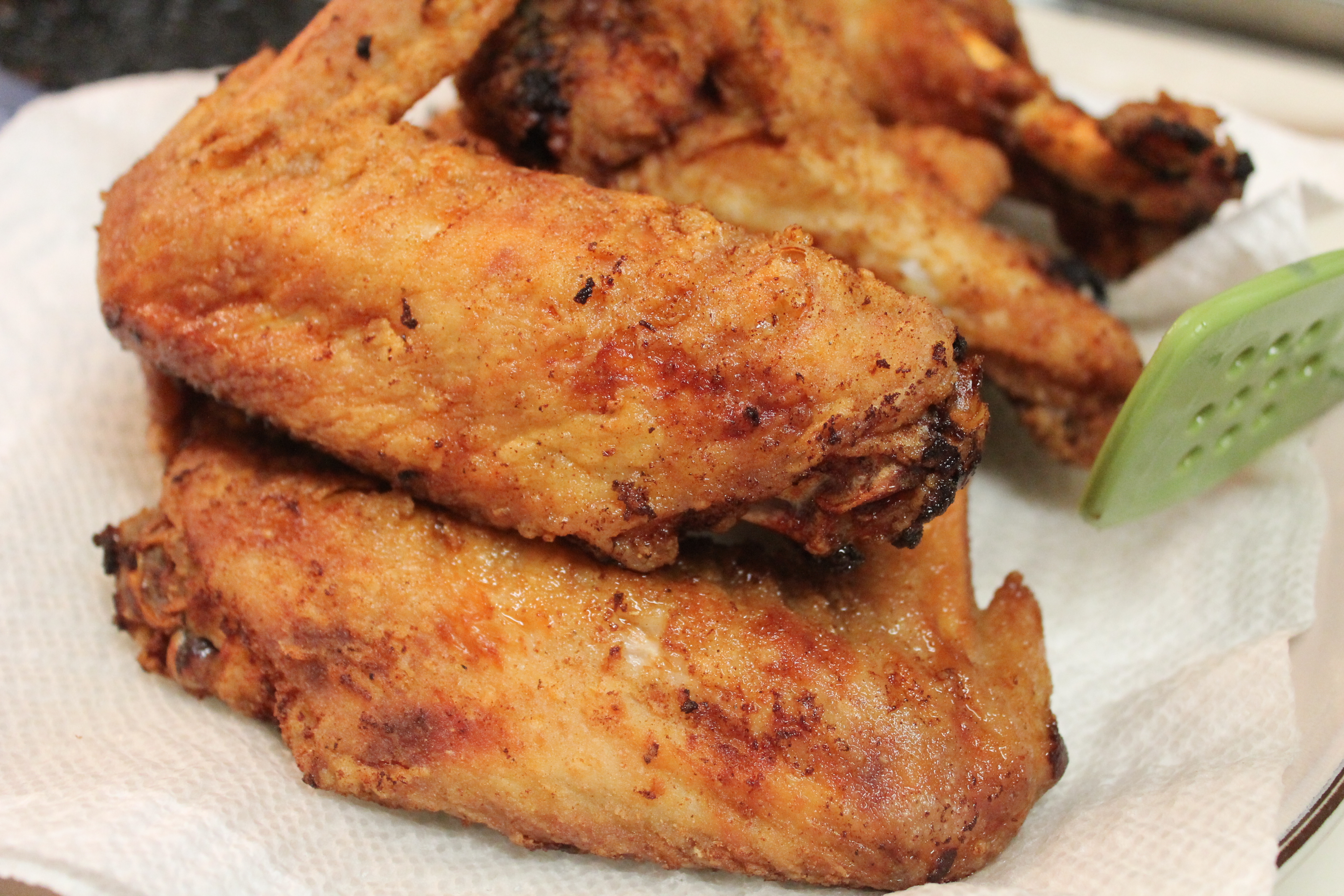The image is a close-up of crispy, fried chicken legs, arranged on a paper towel that rests on a white plate. The chicken skin is golden brown, indicating it has been well-cooked, with a mix of dark brown and blackened areas suggesting a bit of spice but no breading. The chicken legs are stacked, with two pieces prominently in the foreground and two more in the background. A pale lime green kitchen utensil, possibly a spatula with a rounded rectangular shape and several vertical rows of holes, is partially visible toward the right side of the image. The utensil's bright color contrasts with the crispy, oily texture of the chicken and the white background of the paper towel and plate.